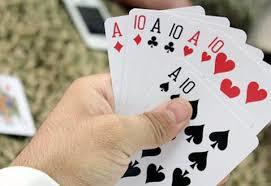In this photograph, the focal point is a person's left hand holding a fanned-out set of playing cards. The background is slightly blurred, though a beige and black-speckled table and an iPhone can be discerned. On the table, there's also a single playing card visible. The person is wearing a long white shirt, with the cuff of the sleeve clearly visible at the wrist. The hand is holding a sequence of aces and tens from each suit. Starting from the left, the cards display are the Ace and Ten of Diamonds, Ace and Ten of Clubs, Ace and Ten of Hearts, and finally, overlapping the Hearts slightly, the Ace and Ten of Spades. The thumb is prominently placed on the Ten of Spades, anchoring the fan of cards.